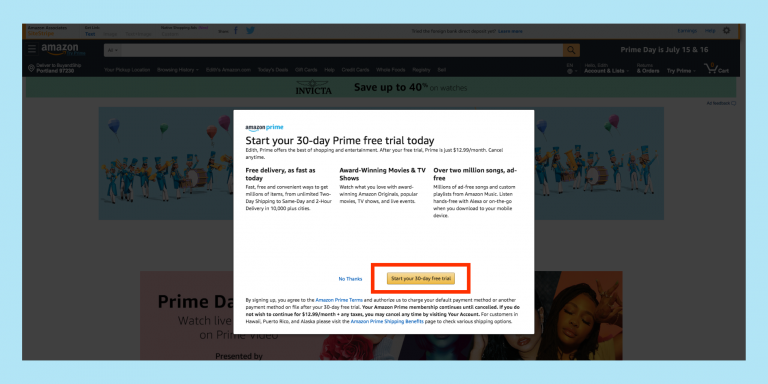The image is a rectangular advertisement featuring a Robin's egg blue border against a blacked-out background. In the center of the ad is a white square that prominently displays the Amazon logo, with "Amazon" written in black and the Amazon smile underneath it, followed by "prime" in blue. Below the logo is the message: "Start your 30-day Prime free trial today" in black print, though the line beneath this text is too light to read. 

The ad emphasizes the benefits of Amazon Prime in three columns:
1. "Free delivery, as fast as today"
2. "Award-winning movies and TV shows"
3. "Over 2 million songs, ad-free"

Towards the bottom, there is a clickable bar with the option "No thanks" in blue text. Beneath this is a red-outlined box with a white background featuring an orange bar that reads "Start your 30-day free trial." Below this, in very small print, are the terms of service.